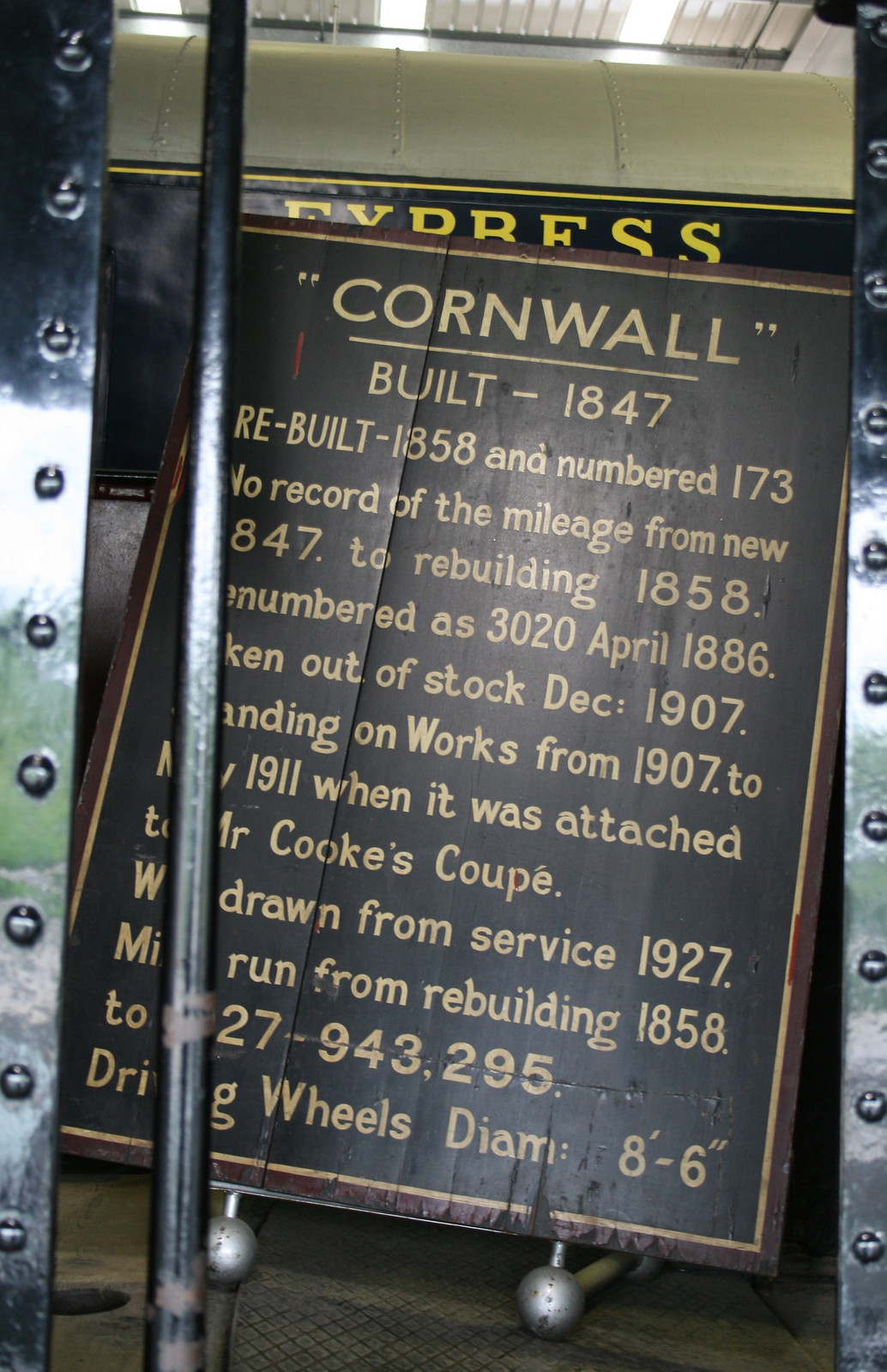The image captures an indoor museum setting, prominently featuring a historical display within a riveted metal case. Central to the display is a brown, possibly wooden sign with tan lettering, partially obscured by a vertical silver pole. The sign meticulously details the history of an item named "Cornwall," potentially a train, dating back to its construction in 1847. The text on the sign reads: 

"CORNWALL, built 1847, rebuilt 1858, and numbered 173. No record of the mileage from new in 1847 to rebuilding in 1858. Renumbered as 3020 in April 1886. Taken out of stock in December 1907. Standing on works from 1907 to November 1911 when it was attached to Mr. Cook's Coop. Withdrawn from service in 1927. 

Near this plaque, there are other metal components and a partially visible sign, with the word "express" discernible in yellow, suggesting a connection to a historical locomotive. Additionally, details indicate variations in wheel diameter, noted as ranging from 8 feet to 8 feet 6 inches."